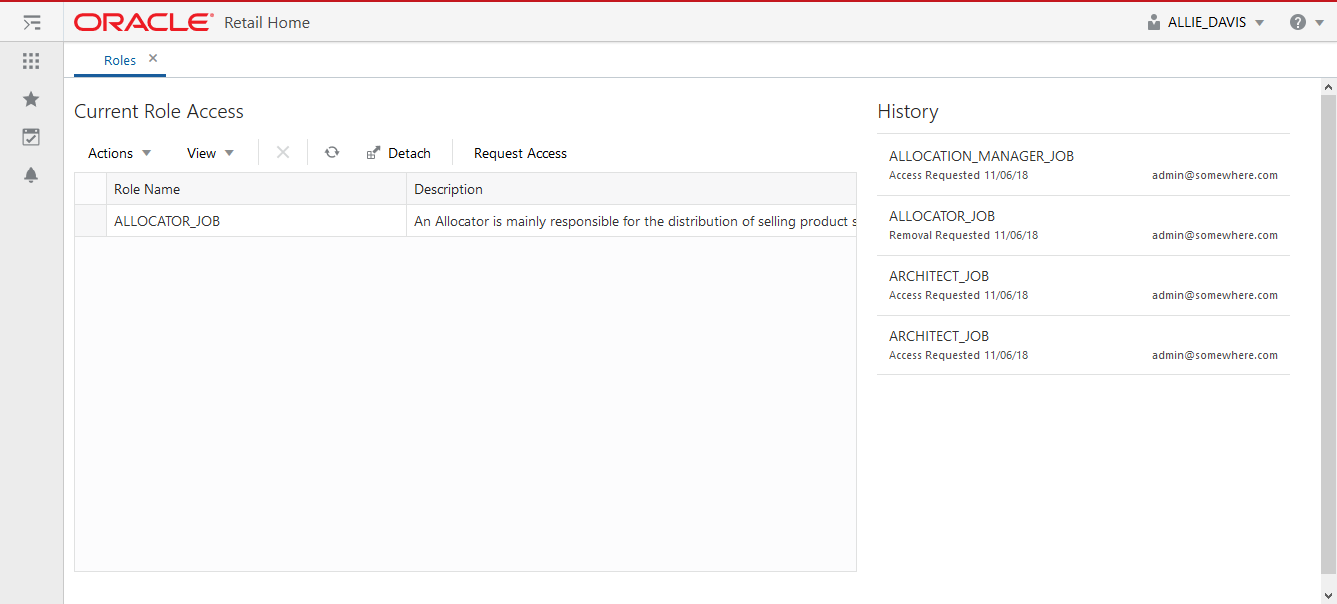In the upper section of the image, a bold red line spans horizontally across the top. On the left side, "Oracle" is prominently written in bold red letters, followed by the word "retail" in gray. Aligning to the right, the text "Allie_Davis" appears in gray, accompanied by two downward-pointing gray triangles, a gray circle with a white question mark inside, and another downward-pointing gray triangle. The background then shifts to white.

In the white background, the word "Roles" is displayed in blue with a capital "R" and is underlined. To its right is a small gray "X". A thin gray line follows horizontally. Below this line, the text "Current Role Access" appears in black, with options "Actions," "View," and an "X" placed alongside two gray circles. Below this, the options "Detach" and "Request Access" are available. 

Further down, the section titled "Role Name" features descriptions like "Allocator_Job", indicating role details. The description beneath states that an allocator is mainly responsible for the distribution of selling products, though part of the text is cut off. To the right, the "History" section lists past actions, including:

- "Allocation_Manager_Job Access requested 11/0A/18"
- "Allocator Job removal requested the same day"
- "Architect Job access requested the same day"
- "Architect Job access requested the same day"

Each action is meticulously documented, showing a history of access requests and role modifications.